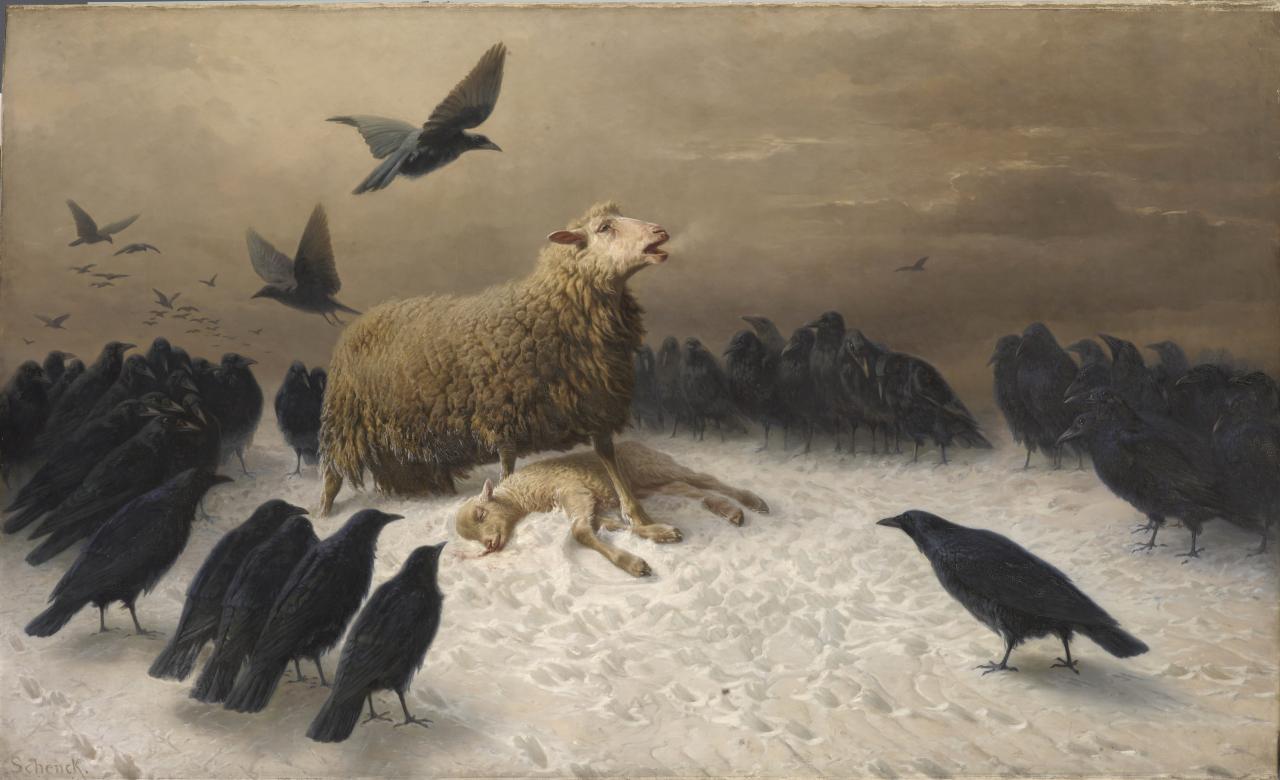The image, possibly a painting or AI animation, depicts a deeply unsettling scene set in a cold, snowy landscape. At the heart of the composition, an older sheep stands over a deceased lamb, likely its offspring, which lies in the snow with its eyes closed and a hint of blood at its mouth. The older sheep appears distraught, its mouth open as if crying out in anguish, expelling visible breath in the frigid air. The color palette of the piece is dominated by muted greys and browns, with a dark, ominous background contributing to the overall somber atmosphere. Surrounding the central figures are numerous black crows, their interest focused intently on the lifeless lamb. Some crows stand on the ground while others circle ominously overhead, heightening the sense of foreboding and despair. The entire scene is permeated by a sense of sorrow and menace, capturing a heartbreaking moment of loss and the relentless passage of nature.